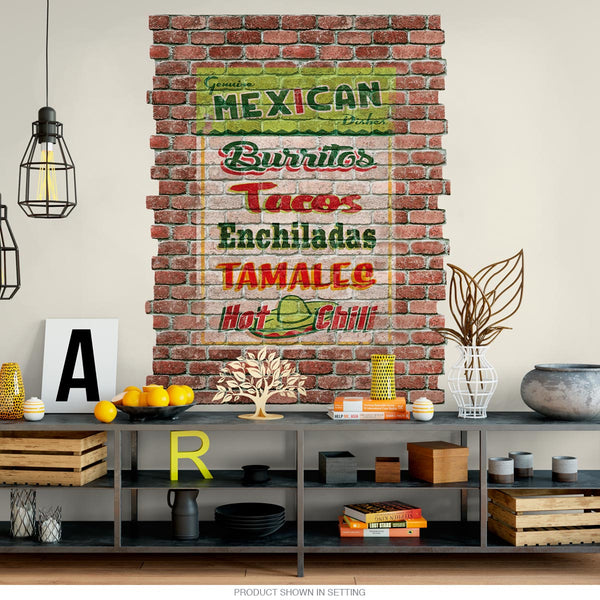The image captures a section of a room dominated by a mural painted with words advertising various "genuine Mexican dishes." The mural, set against a stripe of painted brick wall, prominently displays the words "Mexican" in green at the top. Below this, it lists "burritos," "tacos," "enchiladas," "tamales," and "hot chili," each in alternating colors of green and red. The words "hot chili" are punctuated by an illustrative sombrero between them.

Beneath this mural is an elongated shelving unit, stretching from left to right, brimming with objects. The display includes wooden crates and boxes of varying sizes, pottery, candles, and candle holders. Intriguingly, there's a wire vase adorned with fake wire leaves and several books. Two hanging wire chandeliers shaped like light bulbs add a touch of whimsy.

A significant feature of the arrangement is a prominent, freestanding yellow uppercase letter "R" positioned at the bottom center of the image. On the left side, just above the corner, there's a black plaque featuring a bold uppercase letter "A". The assortment on the shelf also includes lemons, contributing a bright splash of color to the earth-toned display. Additionally, there are metal tree statues, adding a decorative element to the intricate arrangement.